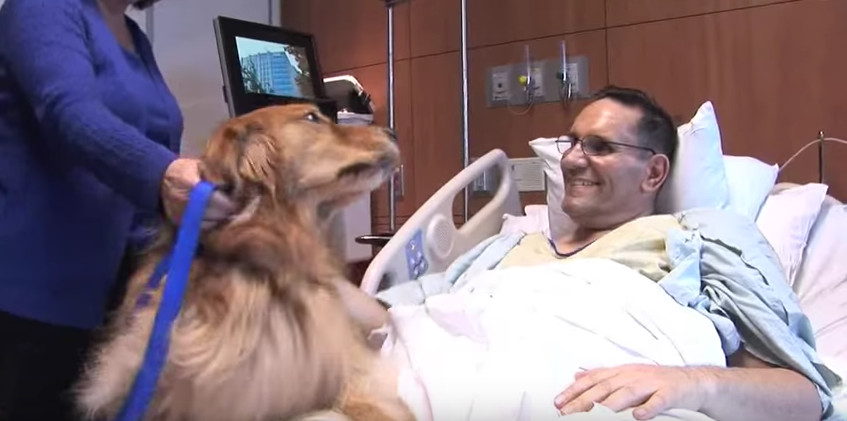This candid horizontal photograph, likely taken with an iPhone, captures a heartwarming moment in a hospital setting. The central focus is a man, around 40 years old, reclining in a bed on the right side of the frame. He is light-skinned, with dark, very short hair, and is wearing black wire-rimmed glasses along with a yellow hospital gown covered by a blue one. He is smiling broadly, showcasing a toothy grin, and looking to his upper left.

A golden retriever with a royal blue leash has its front paws on the man's lap and is turning its head back to look at him, forming an affectionate connection. To the left of the frame stands a woman, whose face is not visible as the image cuts off at her shoulders. Clad in a deep indigo cardigan and black pants, she is holding the dog’s leash. The background reveals a hospital monitor displaying an external view of the building, along with brown and white walls and visible pipes, providing context to the indoor setting. This touching scene exemplifies a therapeutic visit, capturing a shared moment of joy between the man, the dog, and the woman.